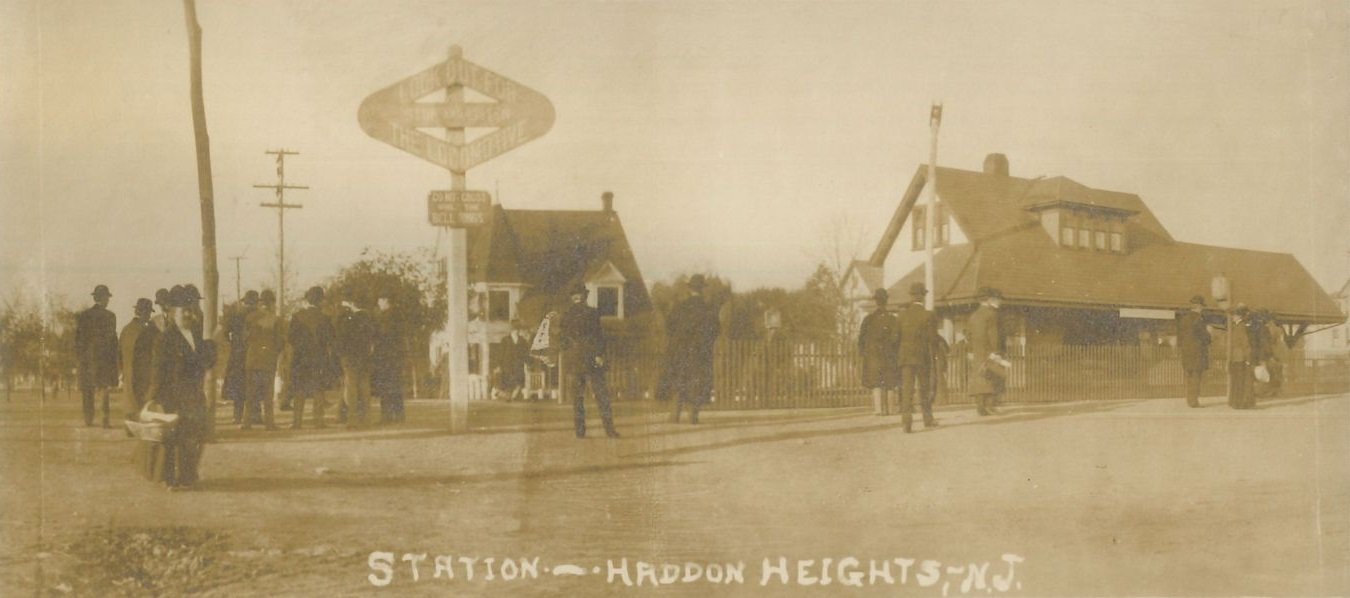This sepia-toned postcard photograph commemorates the opening of a train station in Haddon Heights, New Jersey, around the turn of the 19th to 20th century, distributed in 1907. The image captures a wide-angle view of a dusty, unpaved street where about a dozen men, dressed in turn-of-the-century garb with black round hats, suits, and coats, mill around, possibly awaiting the arrival of a train. The photograph, though faded and not very sharp, reveals two main buildings: a small house and the train station to its right. Off in the distance, on the left, electric or telegraph poles stand, along with some sort of advertising or welcoming sign for the new station. Handwritten in white letters at the bottom of the image is the inscription "station - Haddon Heights, N.J." This vintage photograph, though blurred and worn, provides a nostalgic glimpse into the early 20th-century life of this small New Jersey town.